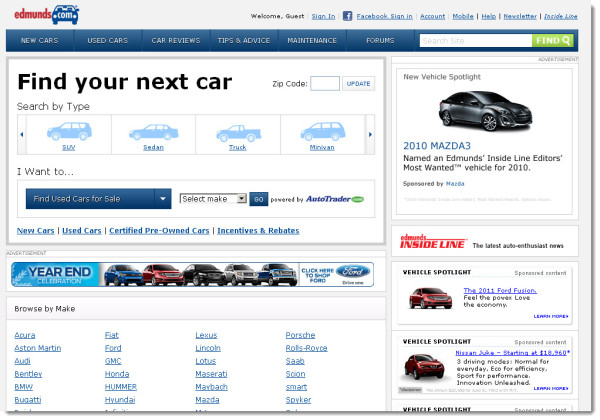Explore Your Next Car on Edmunds.com

In the upper left corner of the image, a prominent text reads "Find Your Next Car." Above this, in the upper right corner, the Edmunds.com logo is displayed. The logo features "Edmunds" in red font, while ".com" is in white font, placed in front of a blue car graphic.

Along the right side of the image, starting from the middle, a user interface section welcomes guests with options such as "Sign In," "Facebook Sign In," "Your Account," "Mobile," "Help," "Newsletter," and a vaguely visible "Share Ride" option.

A horizontal blue navigation bar is positioned below this section, beginning on the left side of the image. The navigation options include "New Cars," "Used Cars," "Car Reviews," "Tips & Advice," "Maintenance," and "Forums." To the right of these options is a white search bar labeled "Search Site," accompanied by a green "Find" button.

The largest font on the image, displayed in black on a white background, reiterates "Find Your Next Car." Beneath this, "Search Types" is listed, with vehicle categories in a horizontal row including SUV, Sedan, Truck, and Minivan.

To the right of the "Find Your Next Car" text, there is a section to enter a zip code, with a data field and an "Update" button. Below this, a dropdown menu labeled "Find Used Cars for Sale" allows users to select a car make, followed by a blue "Go" button. This section is indicated as being powered by AutoTrader.

Further down, an additional navigation menu offers quick links to "New Cars," "Used Cars," "Certified Pre-Owned Cars," and "Incentives & Rebates."